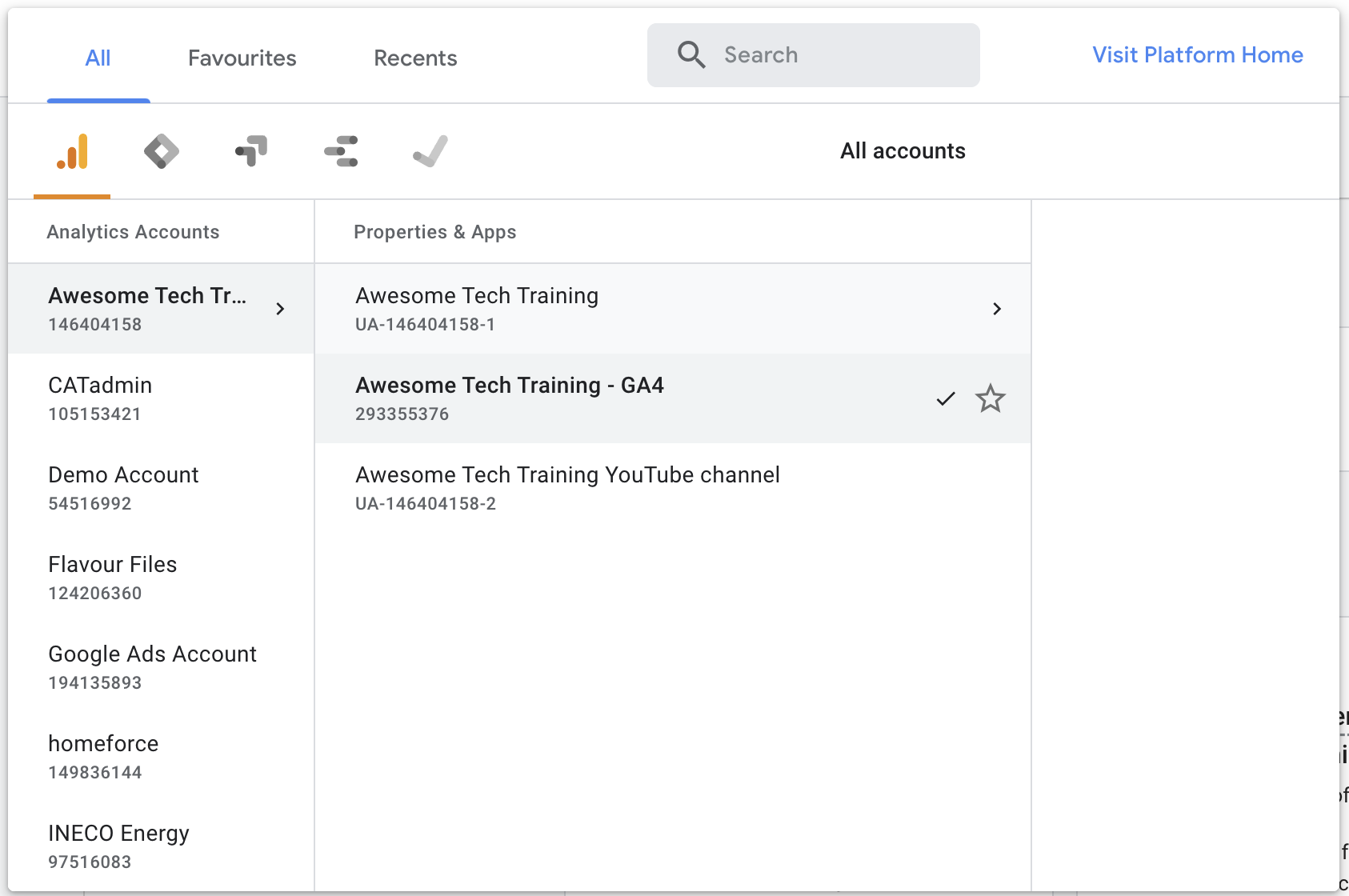The image displays a printout on a white background featuring an interface layout. At the top, there are headings labeled "All," "Favorites," and "Recents," with a search bar to the right, containing an hourglass icon in a muted gray color. Highlighted in blue are the options "Visit," "Platform," and "Home," with "All" also underlined and highlighted as if selected.

Below this, a row features three gold bars of varying heights, accompanied by other selectable icons. To the right of these icons, the words "All Accounts" appear. On the left side, a list of options includes: 
- Analytics Accounts
- Awesome Tech, with ID 146404158
- CAT Administration, with ID 105153421
- Demo Account, with ID 54516992
- Flavor Files, with ID 124206360
- Google Ads Account, with ID 194135893
- Home Force, with ID 149836144
- Ineco Energy, with ID 97516083

In the center of the interface, the headings "Properties" and "Apps" are displayed. Underneath, the next line reads:
- Awesome Tech Training (UA146404158-1)
- Awesome Tech Training (GA4)

To the right, a check mark and a star are visible, and beneath "Awesome Tech Training," the ID 2933355376 is shown. Below this, it reads:
- Awesome Tech Training YouTube Channel (UA146404158-2)